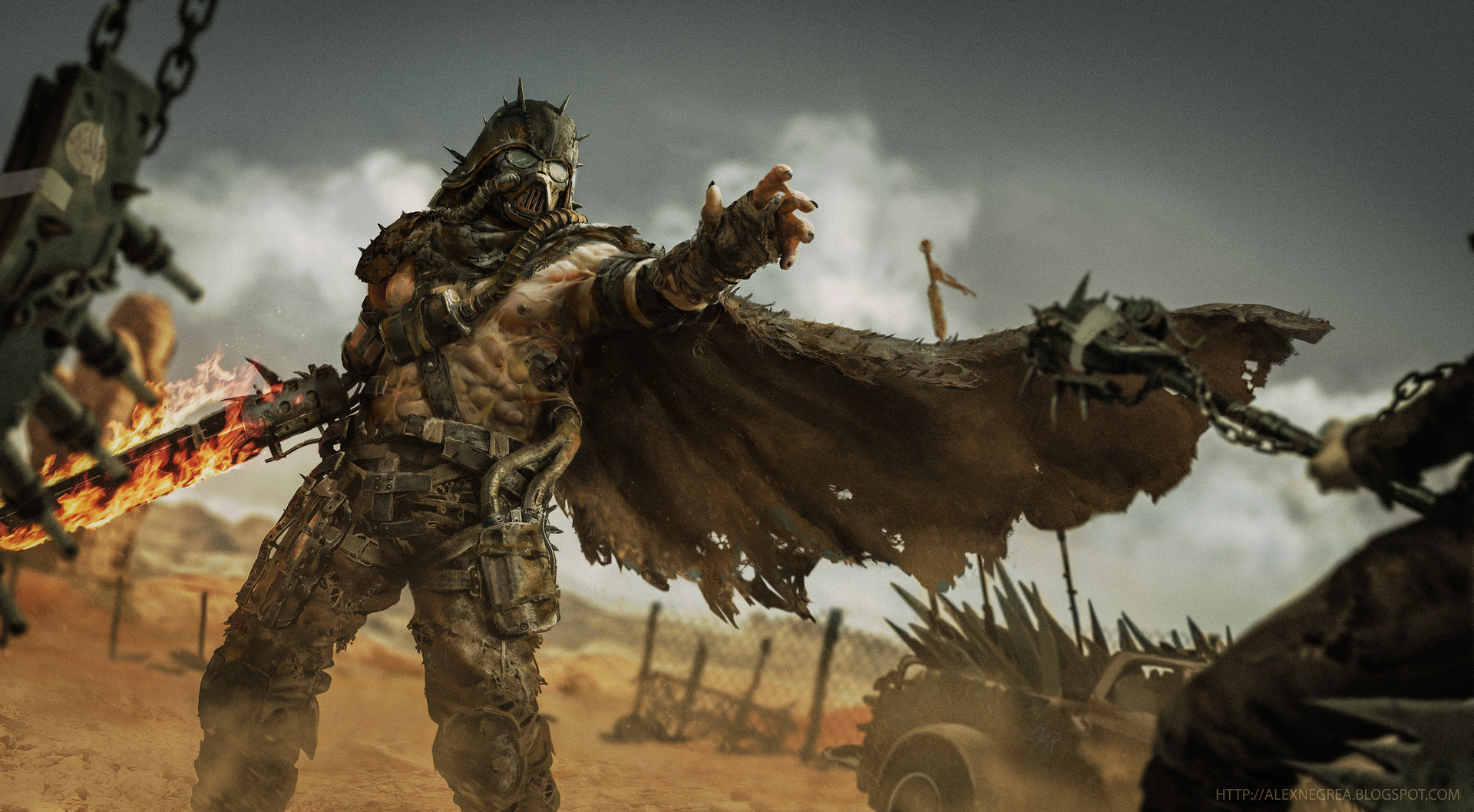In this captivating video game scene, the focal point on the left is a rugged character adorned in heavily worn and deformed clothing, exuding a post-apocalyptic aura. The attire, light gray in color, resembles a blend of dystopian battle armor, featuring numerous small spikes embedded throughout. The character's head is shielded by a helmet crowned with additional spikes, enhancing their fierce appearance. Clutched in their hand is a formidable sword, from which red flames dramatically erupt, adding an intense, fiery element to the scene. A large, tattered cape billows from the character's neck to the right side, amplifying the sense of motion and chaos.

The background further sets the desolate tone with a dilapidated car, rusted and heavily damaged, hinting at past turmoil. Beyond the car, a broken fence extends across the sandy, light orange terrain, emphasizing the harsh, arid desert setting. Above, the sky is a somber shade of gray, dotted with light clouds, casting a bleak atmosphere over the entire scene. This detailed portrayal immerses viewers in a gritty, hostile world, teeming with dramatic and foreboding elements.